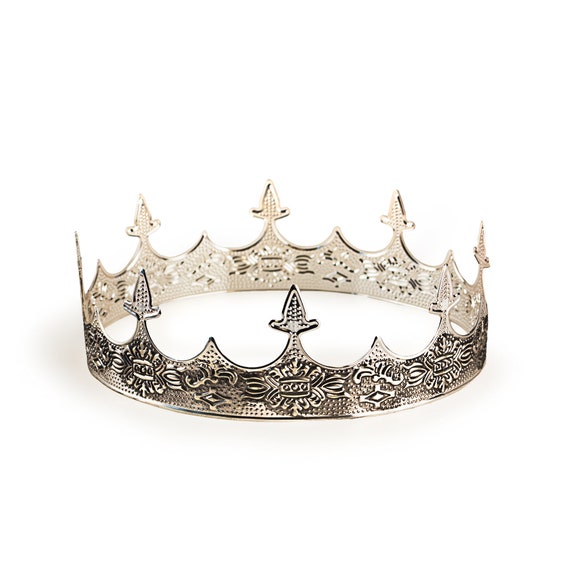This is an image of a crown set against a white background. The crown itself is predominantly silver with ornate, medieval-style engravings and an intricate pattern along its outer border. The design features dots and other fine details, which give it an elegant and royal appearance. The crown also includes eight spearhead-like protrusions that rise in a wave-like pattern, reminiscent of traditional king's crowns. Additionally, there are shades of dark brown or bronze accentuating the engravings and indentations, creating a rich, contrasting texture. The inside of the crown is visible, adding depth to the image. The overall impression is one of regality and craftsmanship.